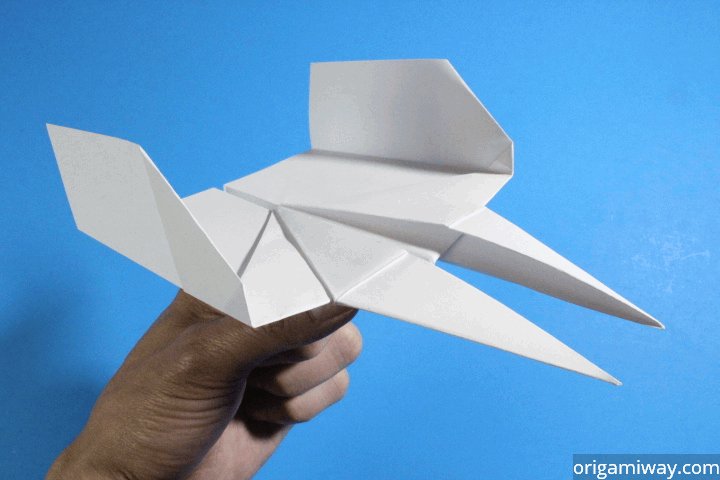In this detailed photograph, a person with dark-toned skin is poised to launch an intricately folded origami airplane made from plain white paper. The unique design features two pointed noses at the front, an open slit running halfway down the center, and diamond-shaped folds. The wings are short, wide, and have small upward-folded flaps, indicative of a carefully crafted model that might remind one of futuristic aircraft seen in 'Star Wars' or 'Star Trek'. The background is a solid, soft blue, and in the lower right corner, the text "origamiway.com" suggests the image is part of promotional material for the origami-focused website. Every fold and crease of the origami is visible, adding to the detailed craftsmanship of this airplane.